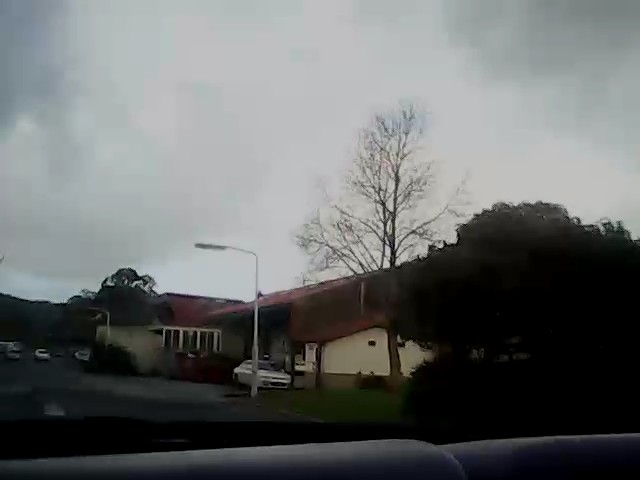This photograph, likely taken from within a car through the front windshield, captures a street scene on a gloomy, rainy day. The image quality is somewhat blurred, potentially due to raindrops. In the foreground, there is a gray dashboard with a black lining visible at the bottom of the image. The sky above is heavily overcast with dark gray clouds, and there is no hint of sunlight penetrating the scene.

The main focus of the photograph is a house with white walls and a red, sloped roof positioned slightly to the left. In front of the house, a white car is parked. There's a prominent metal pole with a streetlight and some curved white streetlights can also be seen. On the right side of the image, there is a substantial green tree, full of leaves, juxtaposed against a tall, barren tree with a narrow trunk, devoid of leaves, which suggests it could be winter.

Further along the road, which extends beyond the car, a few distant cars are visible, indicating traffic in the area. Another house with similar red roofing and yellow siding is partially visible next to the main house. The overall scene is characterized by the stark contrast between the lush green tree and the leafless barren tree, the wet, reflective street, and the somber, cloud-covered sky, painting a vivid picture of a rain-soaked, dreary day.